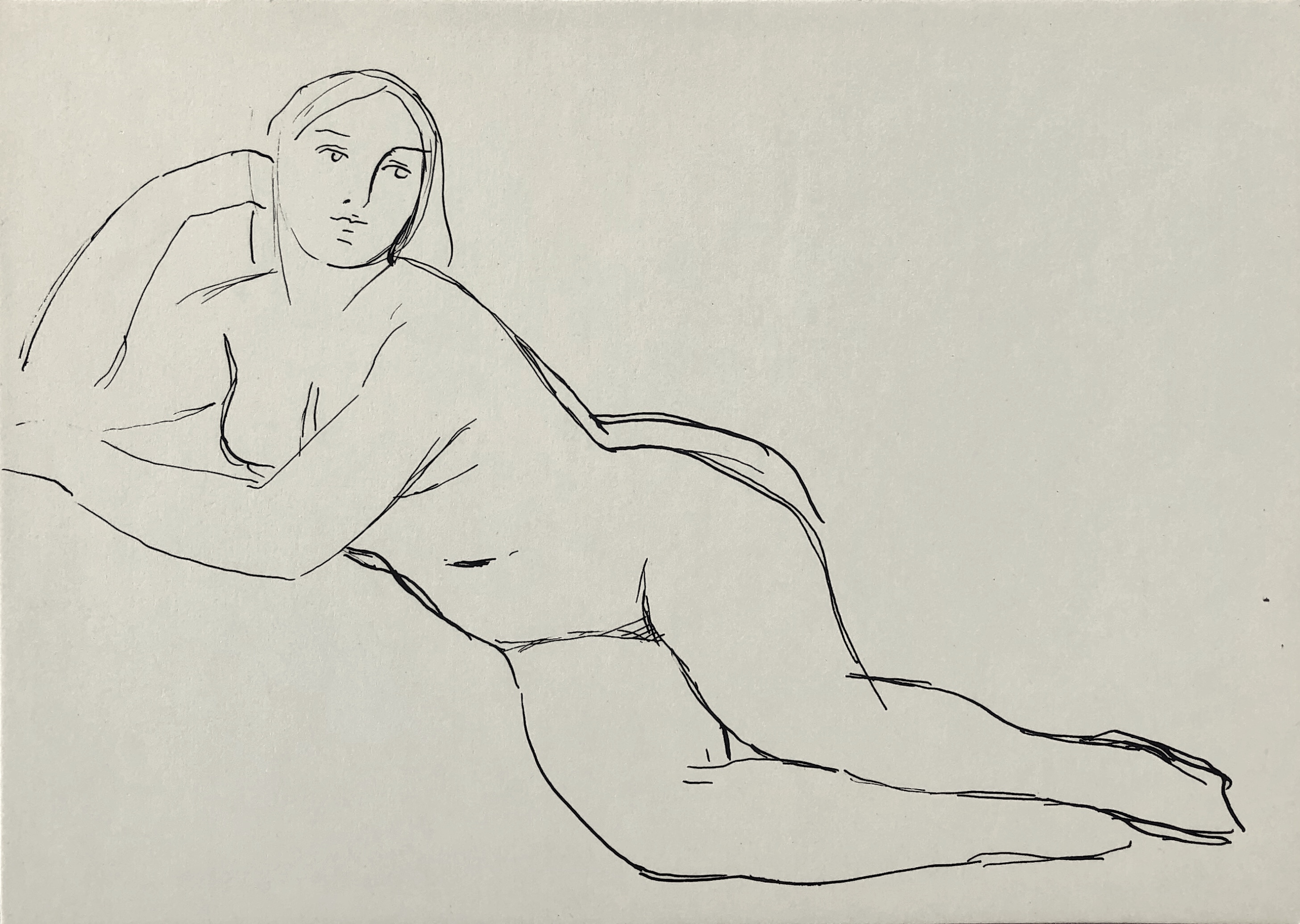The image is a black-and-white pencil line drawing on a textured, slightly grayish-white paper background, depicting a nude woman lying on her right side. She has a prominently round face and body, with distinct facial features, including a very prominent nose that almost overlaps her right eye. The woman has medium to long hair cascading over her shoulders and is gazing over her right shoulder towards the viewer. Her right arm is bent with her hand curled behind her head, resting against her cheek, while her left arm extends beneath her right elbow and curves to cover her breast. Her legs are together with toes pointed, and her body is outlined in black lines, suggesting movement and form, with additional lines running down her back and lower back, possibly hinting at clothing or shadow but otherwise depicting her nude form. She appears to be leaning on an unseen surface, perhaps the edge of a sofa or pillow, creating an intimate and relaxed pose. The minimal background and rough sketch style emphasize the simplicity and rawness of the artwork.